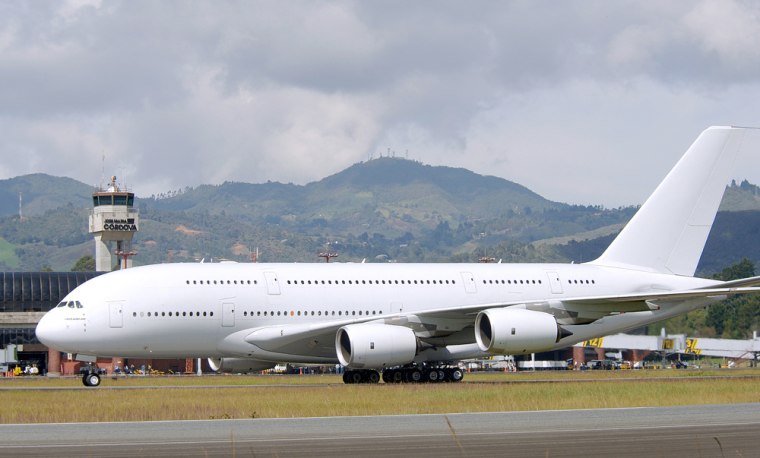The image depicts a large, white, four-engine double-decker jet parked at an airport. The jet is stark white with no visible markings or logos. It features two rows of windows along its fuselage, indicating its double-decker design, and has a small cockpit at the front. The plane's wings have two engines each, making a total of four propellers. The airport setting includes an air traffic control tower in the background with the visible letters "Cordova." The scene is well-lit, suggesting daylight, and the sky is filled with gray, ominous clouds. In the background, verdant mountains covered in greenery rise up, hinting at a moisture-rich environment. Beneath the plane, cars, luggage, and airport equipment are visible, adding to the bustling atmosphere of the location. Overall, the image captures a detailed and dynamic airport scene with a prominent, unmarked aircraft.